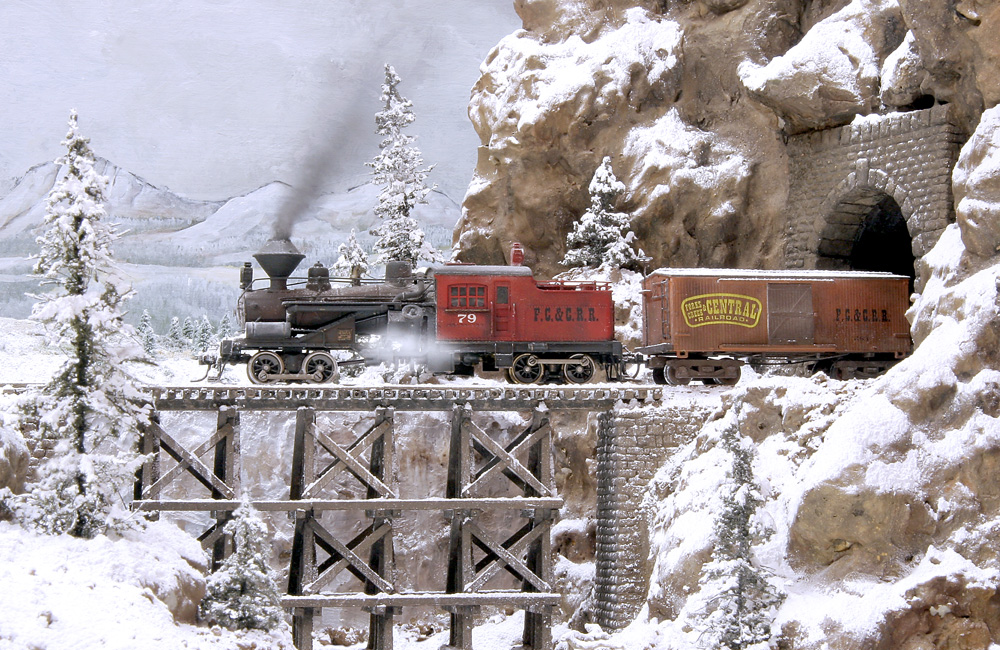In a beautifully detailed winter scene, a miniature train set captures the essence of an older era with meticulous craftsmanship. The backdrop features snow-covered mountains with detailed fine black outlines and a primarily white sky, punctuated by some clouds. Tall trees laden with snow frame the image, adding depth to the snowy mountain outlook.

At the center of the scene, a steam engine train, designed in an old claymation style, emerges majestically from a tunnel carved into a rocky mountain. The black engine leads the spectacle, puffing clouds of smoke from its stack. Trailing directly behind is a red carriage labeled with the number 79, understood to be the engineer’s quarters, distinguishable by large letters "FC and CRR."

Following the engineer's car, a longer, slightly duller brown carriage comes into view, marked with "Central Railroad" in yellow lettering and also bearing the "FC and CGR" logo. The train traverses an older, intricate wooden bridge with numerous supports as it makes its journey from right to left. Layers of snow enhance the bridge and the foreground, complementing the serene, frozen lake nestled in the valley below the majestic snowy mountains in the background.